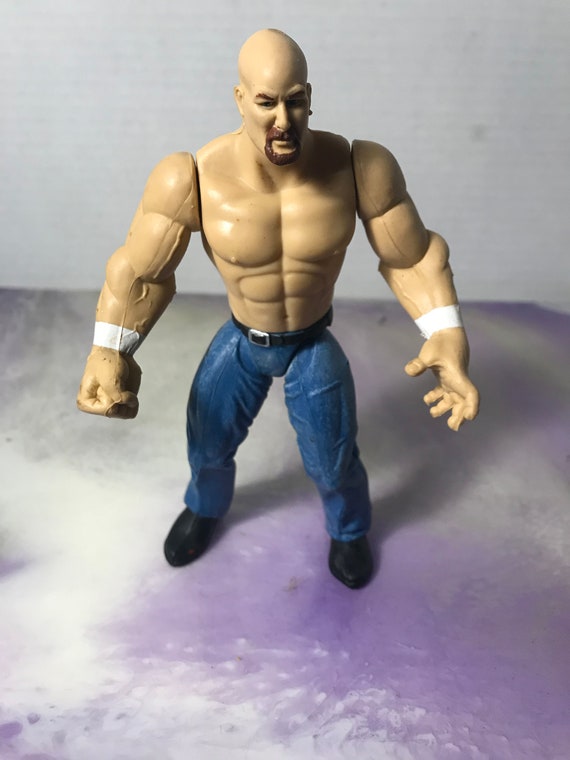In this image, there is a highly detailed plastic action figure of a muscular male, resembling a wrestler. This topless figure is bald with a brown goatee and sports two white wristbands. The doll's impressive physique showcases defined muscles, including his back, abs, shoulders, biceps, triceps, and forearms. He is dressed in painted blue jeans, fastened with a black belt, and wears black shoes. His left hand is partially clenched, while his right hand is clenched into a tight fist. The toy is standing on a purple and white, uneven, bumpy surface, and the backdrop features a dirty white background with a noticeable stain on the right side.